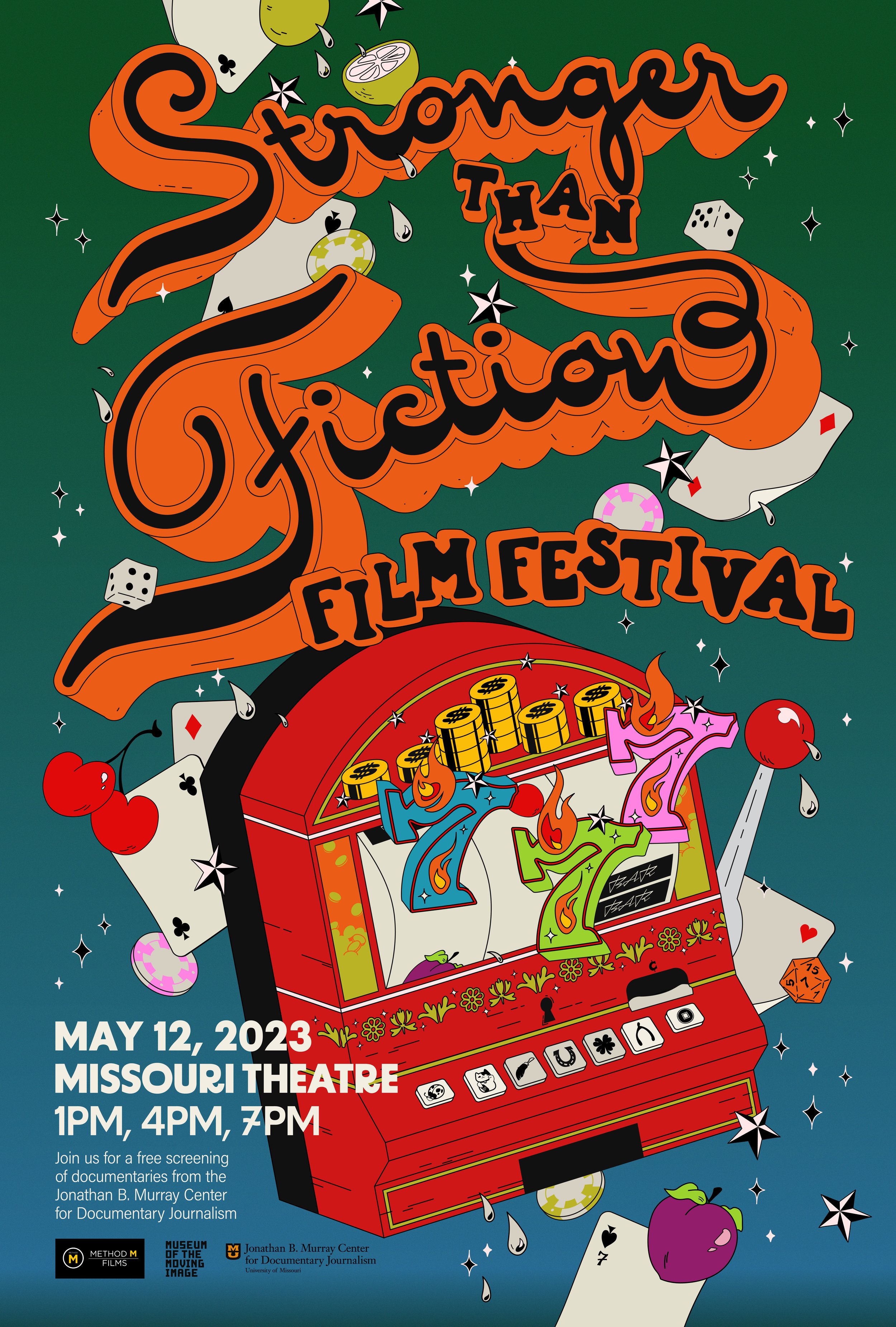The poster advertises the Stranger-Than-Fiction Film Festival, featuring a vibrant, stylized design. It prominently displays a cartoon-style slot machine showing a lucky 777 in blue, green, and pink, with symbols and buttons--two of which have distinct logos. The machine's handle is red with a white lever, and playing cards and dice add to the casino theme. The background transitions from green at the top to blue at the bottom. The text is heavily stylized in black and red-orange. In the lower-left corner, details in white text announce the date and venue: May 12, 2023, at the Missouri Theatre, with screenings at 1 p.m., 4 p.m., and 7 p.m. Attendees are invited to a free screening of documentaries from the Jonathan B. Murray Center for Documentary Journalism. Logos for various institutions are included, emphasizing a collaborative event.